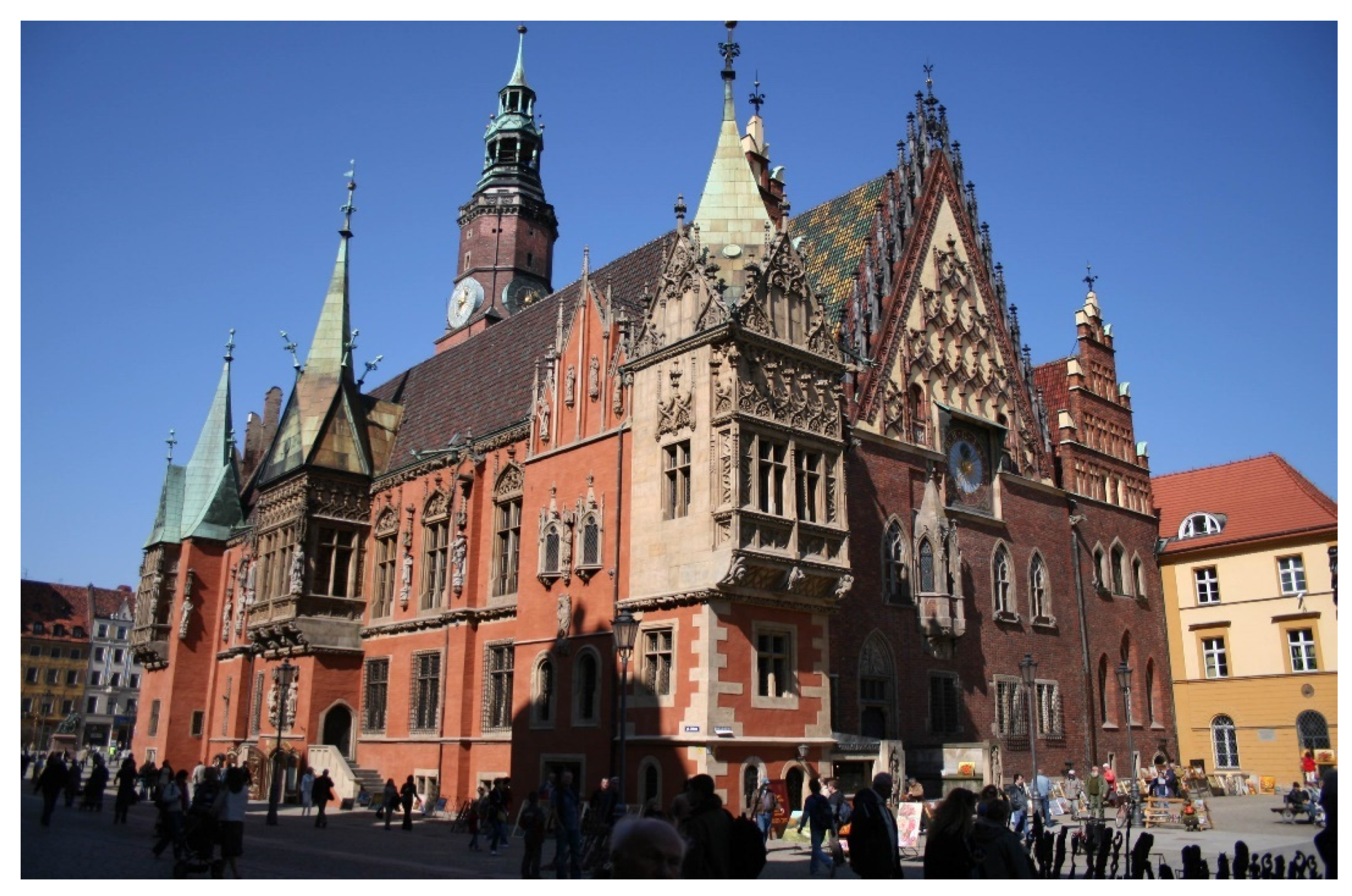This photograph captures an old, intricately designed cathedral, likely of European origin, displaying a vivid and colorful facade with dominant shades of red, brick, and beige. The building is characterized by its numerous ornate windows and multiple peaks and spires, including a blue-topped tower that adds to its striking appearance. The side of the building we face in the image features a light red exterior with a variety of intricate architectural details, while the rear displays additional peaks and a prominent clock tower perched at the top. The cathedral is set within a bustling city environment, surrounded by buildings with complementary tans, whites, and red shingle roofs. A crowd of people is seen milling around the cathedral, suggesting it is a well-frequented yet not overly touristy location. The overall atmosphere of the image is one of historic grandeur, captured amidst an everyday urban scene.